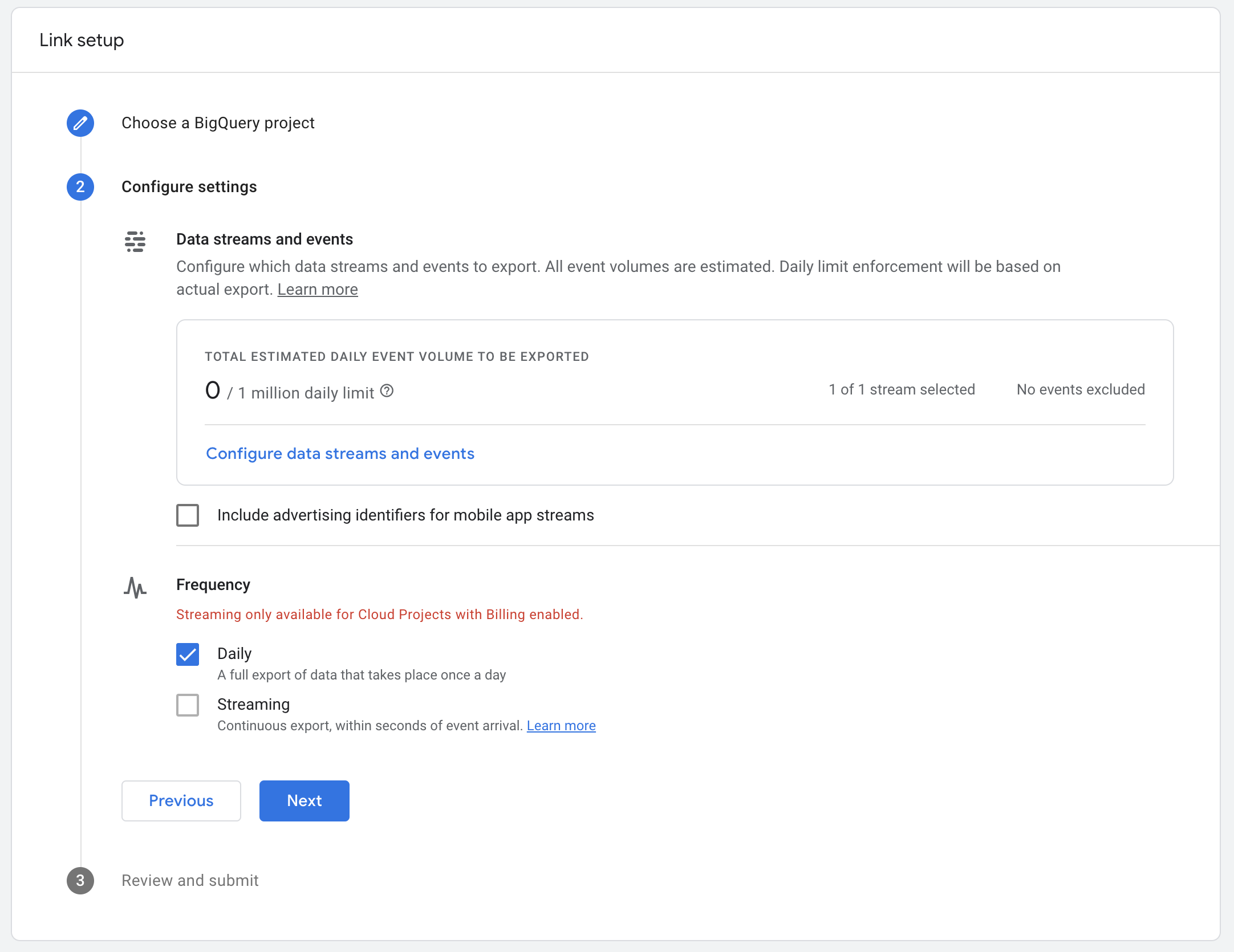**Detailed Descriptive Caption:**

This image displays the link setup page for an application. In the upper left-hand corner, the title "Link Setup" is prominently visible. The page is primarily composed of textual information, checkboxes, and instructional headings.

The first section instructs users to "Choose a Big Query Project." Following this, the "Configure Settings" section appears, encompassing options titled "Data Streams and Events." Users are guided to configure which data streams and events they wish to export. A note indicates that all event volumes are estimated, and daily limit enforcement will be based on actual exports, with an accompanying "Learn More" hyperlink.

Further down, an option labeled "Total Estimated Daily Event Volume to be Exported" is displayed, marked as "Zero of one million, the daily limit." Below it, a status reads "One of one stream selected, no events excluded." There's a checkbox beneath this that allows users to "Include Advertising Identifiers for Mobile App Streams."

The "Frequency" section follows, featuring a warning in red text that reads "Streaming Only Available for Cloud Projects with Billing Enabled." Users can choose between two options via checkboxes: the first checkbox, marked "Daily," indicates a full data export occurring once a day and is checked by default. The second, unchecked option, labeled "Streaming," denotes continuous export within seconds of event arrival and includes a "Learn More" hyperlink.

At the bottom of the page, navigation options for "Previous" and "Next" are provided. The final piece of text on the screen states "Number three, Review and Submit," indicating the subsequent step in the setup process.